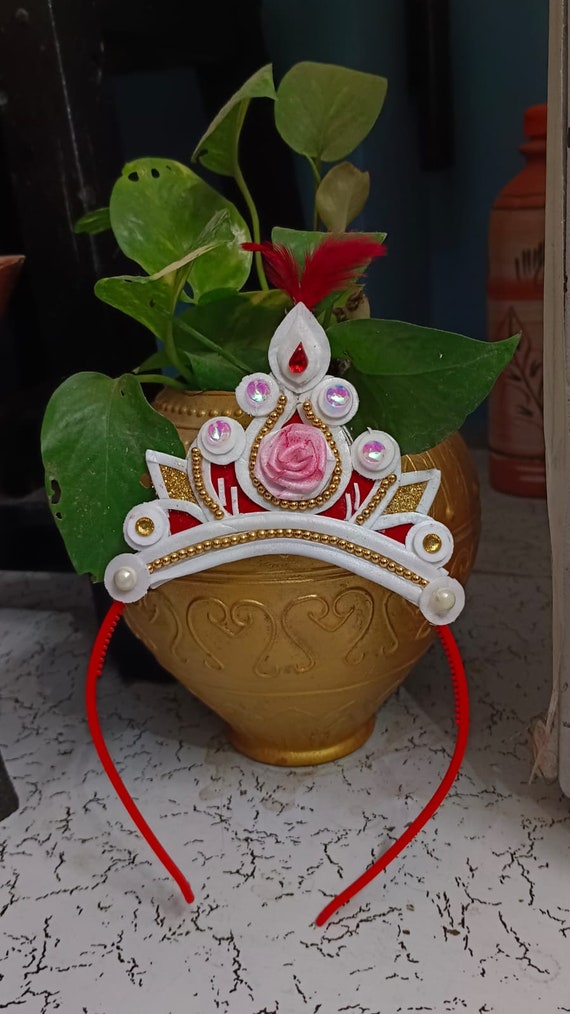In this detailed image, a potted plant with large, slightly damaged green leaves sits in a gold-colored planter, set on a white floor. Leaning against the planter is a distinctive, girly headband resembling a tiara. The headband itself features a red band, with an ornate section rising from its center. This section is adorned with intricate white and gold roping and a plethora of gems, including white pearls, yellow, purple, and red jewels. Central to this decorative array is a vivid pink rose. The headband's design, combined with the luxurious gold planter, creates a charming indoor scene.